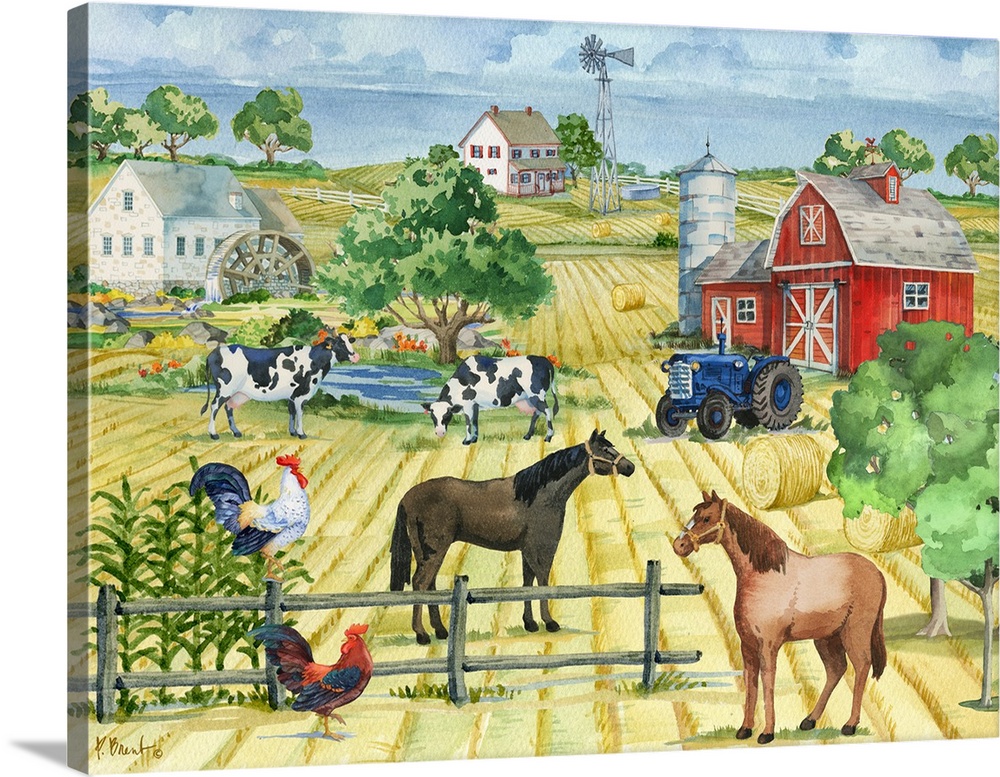This detailed painting on a thick, slightly cantered canvas depicts a vibrant farm scene. In the foreground, two horses—a light brown one and a dark brown one—stand to the left and right among vertical lines of hay that stretch back to the horizon. To the left of the horses, a red and black rooster and a white and black rooster stand near a small brown fence with four posts and four corn stalks growing between them. The background features two black and white cows and a blue tractor. Further back, a large red barn with a silo is seen to the right, while a white house with a water wheel and a small pond occupies the left side. Far in the distance, a two-storied white farmhouse with an adjacent windmill completes the pastoral landscape, bordered by trees and expansive fields. The painting, done in a folk art watercolor style, wraps around the edge of the canvas, capturing the essence of rural life.